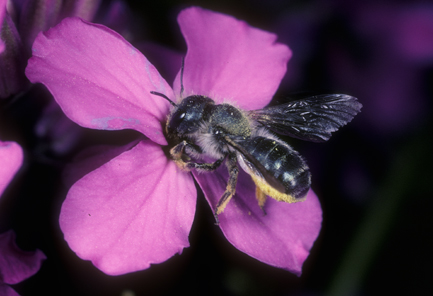In this highly detailed and close-up image, a bumblebee is seen pollinating a pinkish-violet, four-petaled flower, possibly a violet or an iris. The background is predominantly dark, with hints of green leaves, creating a striking contrast. Dominating nearly an entire petal, the bee features a large black head with two black antennae and dark eyes, with its side appearing slightly grayish. The bee’s body exhibits a distinct pattern: primarily black with fuzzy textures, thin white lines, and yellow edges. Its legs are also fuzzy, with the top parts being black and the lower sections displaying a mix of black and yellow. The bee’s translucent wings are folded at rest, and its bean-shaped body reveals its vibrant coloration, including a yellow, fuzzy underside. The intricate details of the bumblebee’s anatomy are sharply highlighted against the soft petals of the flower it diligently pollinates.